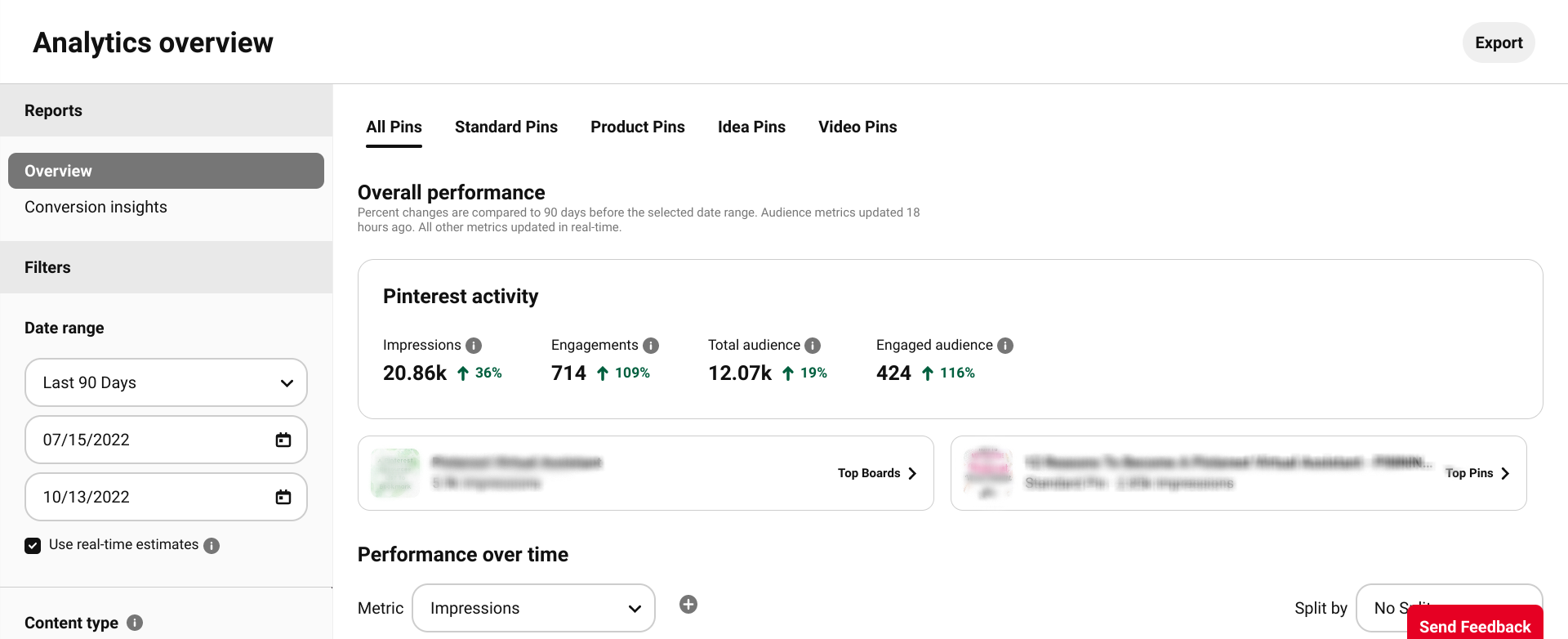The image displays a detailed webpage from an analytics dashboard. At the top, the heading "Analytics Overview" is prominently featured in a bold black font. Below it, there's a gray navigation bar with the options labeled "Reports" (selected and in a darker gray), "Overview," "Conversion," "Insights," and "Filters."

The selected date range is "Last 90 days," with a dropdown menu available for further customization. The specific dates from "07-15-2022" to "10-13-2022" are highlighted. A black checkmark box is present, indicating the option "Use real-time estimates."

In bold black font, "Content Type" is listed with categories such as "All Plans," "Standard Plans," "Product Plans," "Idea Pins," and "Video Pins."

The next section titled "Overall Performance" displays various metrics under the subheading "Pinterest Activity." It shows:
- Impressions: 20.86k
- Engagements: 714
- Total Audience: 12.07k
- Engaged Audience: 424

All metrics are accompanied by green arrows, signifying spikes in traffic. Additionally, there's a "Performance Over Time" graph with the metric currently set to "Impressions," featuring an adjustable dropdown menu to change the displayed metric.